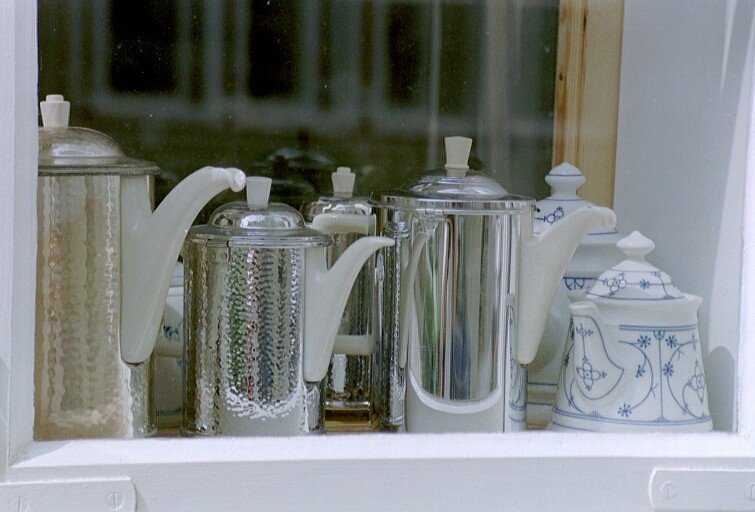The image showcases a collection of coffee or tea pots elegantly arranged on a white shelf. On the left, the largest pot has an aged patina and a hammered silver finish, contrasted by its white ceramic spout and knob. Immediately to its right is a slightly shorter pot with a similar hammered texture but a shinier and cooler silver finish, also featuring a white ceramic spout and knob. The next pot, a tad larger than the previous one and with a smooth silver finish, also includes white ceramic details. On the far right, a distinctive white porcelain pot adorned with a blue line design stands out. The shelf is positioned in front of a reflective surface, possibly glass, framed by bare wood trim visible on the right. White painted brackets are seen in the lower corners, supporting the shelf, which may be part of a cabinet structure.